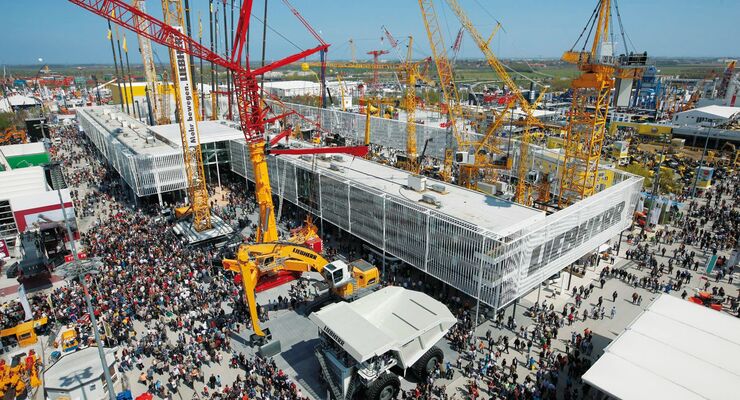This aerial daytime image captures a bustling construction site at an industrial location, possibly a factory or event display. Dominated by clear blue skies, the scene centers around a predominantly white building, featuring black lettering spelling "Lieber" on its side. An assortment of construction machinery, including tall yellow and red cranes, surrounds the building. There's a noticeable large white crane with black windows on the left, and a prominent white piece of machinery with black lettering on the visor to the left. A white flat-roofed structure is visible in the lower right corner. The construction area is filled with a vibrant array of colors including yellow, orange, white, red, blue, green, and silver. The site teems with people, standing and possibly assisting with the construction or simply observing the activity. The angle and scale suggest this is a significant construction event, viewed from above.